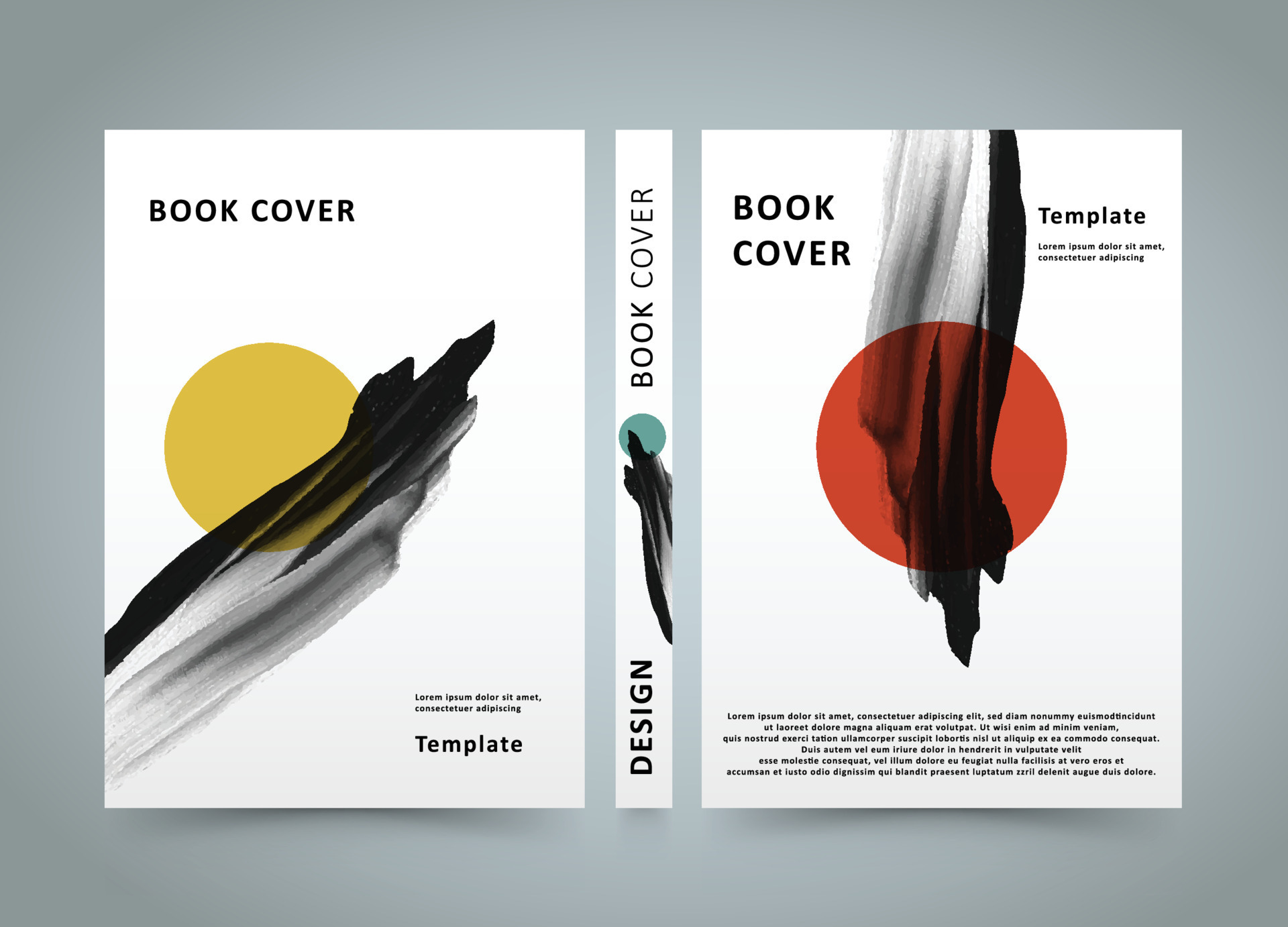This image showcases a conceptual design for a book cover, displayed as if the book is laid open to reveal its front, spine, and back sections. The background is a subtle gradient of silver-gray, accented with white highlights around the center. Each section maintains a cohesive theme with a light off-white background and distinct circular elements.

On the left, representing the back cover, the top left corner features the text "book cover" in black. The centerpiece is a golden yellow circle with a black and gray smudge over it. At the bottom right, placeholder text reads "Lorem Ipsum Dollar Sit Emet Constrictor Adepising," followed by the word "template."

The spine, located centrally, carries the title "design" vertically at the bottom, with "book cover" at the top. It displays a greenish-blue circle mottled with a black paint splash in the middle.

The right section represents the front cover, mirroring the structure of the back. It carries "book cover" in the upper left and "template" in the upper right corner. Dominating the center is a reddish-orange circle imbued with a black and gray smudge. A faint paragraph of placeholder text is visible at the bottom, though it is too small to be legible.

Overall, the design uses consistent visual elements and typography to deliver a balanced, modern aesthetic for a book cover template.